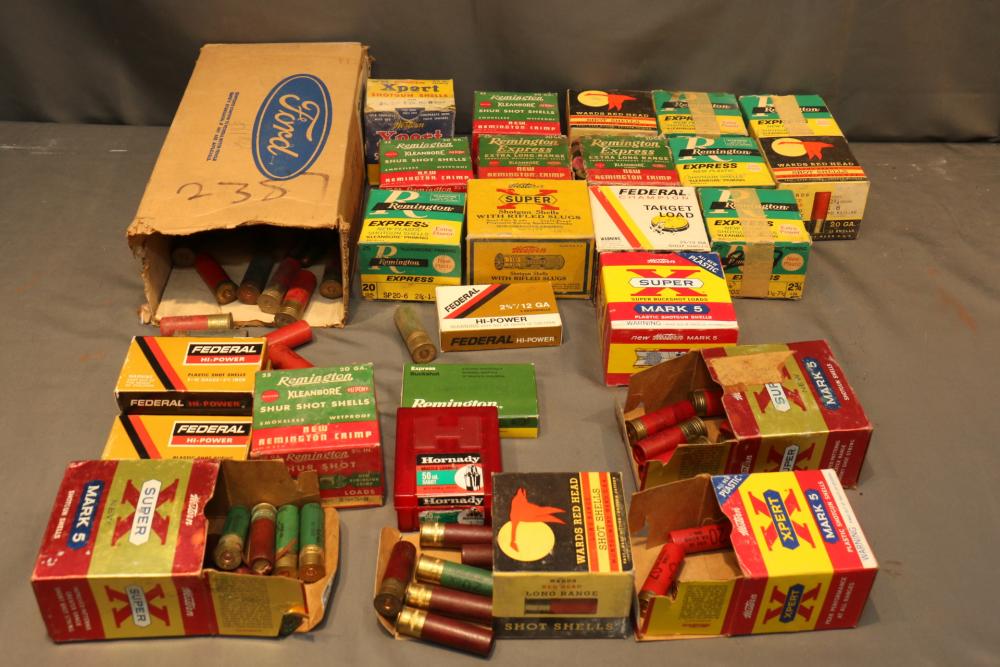The photograph, taken indoors under artificial light and clearly staged, depicts a carefully arranged collection of shotgun ammunition. The composition is square with no border, featuring a muted gray canvas as both the surface and the background. Dominating the upper left corner of the image is a large, plain cardboard box branded with the blue Ford logo and the markings "2357." This open box is overflowing with shotgun cartridges, primarily maroon, green, and red, each with brass tips.

Surrounding the larger box are numerous smaller boxes, varying in size and brand, but predominantly colored in shades of green, yellow, and red. While most of these smaller boxes are closed, several are open, revealing their contents spilling out. The cartridges scattered around match the hues found in the large box – rich reds, greens, and some yellow tones. The assortment of boxes and cartridges rests on the gray cloth, with the backdrop of a slightly darker gray canvas enhancing the vivid colors of the ammunition.